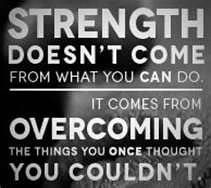This low-resolution, small square image features a wavy black and gray, cloudy background. The image is devoid of any borders and predominantly showcases a motivational quote in light gray, all-caps text with a faint gradient. At the top, the quote starts with the word "STRENGTH" in very large letters, followed by "DOESN'T COME" in slightly smaller letters, and "FROM WHAT YOU CAN DO" in the smallest size yet. Separating the two halves of the quote is a distinct white horizontal line. Below this line, the text resumes with "IT COMES FROM" in the smallest letters, "OVERCOMING" in larger text, and finally, "THE THINGS YOU ONCE THOUGHT YOU COULDN'T" in slightly larger letters than the previous line. Though pixelated, this inspirational message is designed to uplift and is likely intended for social media sharing.